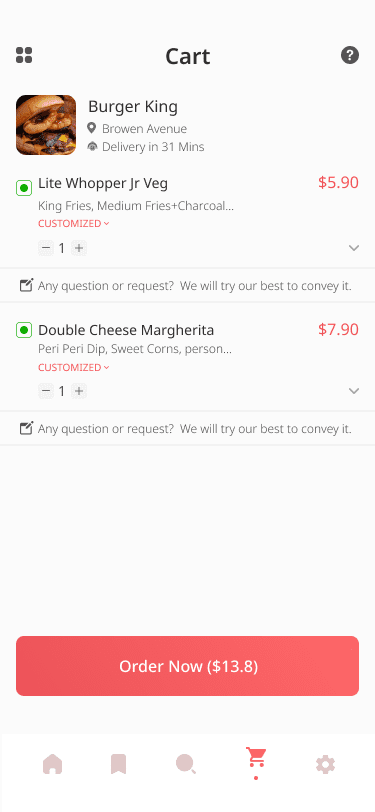The image displays a food ordering app interface on a mobile device, possibly a phone or tablet, reminiscent of services like Uber Eats. The app screen features a minimalist design on a white background. In the top left corner, there is an icon comprised of four small squares forming a larger square. Centrally, the word “Cart” is displayed in dark grey, accompanied by a dark grey circle with a white question mark in it on the far right.

Below this header, there is a vivid picture of a mouth-watering burger, showcased in profile. The burger is stacked with massive onion rings, slathered in a reddish-brown sauce, containing a juicy beef patty, a slice of cheese, and cushioned by two white burger buns. To its right, the text reads “Burger King,” along with the delivery location “Browen Avenue” and an estimated delivery time of 31 minutes.

The user has selected items including a “Light Whopper Junior Veg,” a “King Fries,” and “Medium Fries plus Charcoal…” The price for this selection is $5.90, highlighted in red, with a note indicating that the order is customized. Beneath this, a light grey line provides a message: “Any question or request, we will try our best to convey it.”

Another order item listed is a “Double Cheese Margarita,” “Berry Berry Dip,” and “Sweetcorns…” This order costs $7.90, also highlighted in red, with customization noted. Another grey message line repeats the assurance about conveying any questions or requests.

At the very bottom of the screen, a prominent red button with white text instructs the user to “Order Now.” The total cost for the selected items is displayed as $13.80.